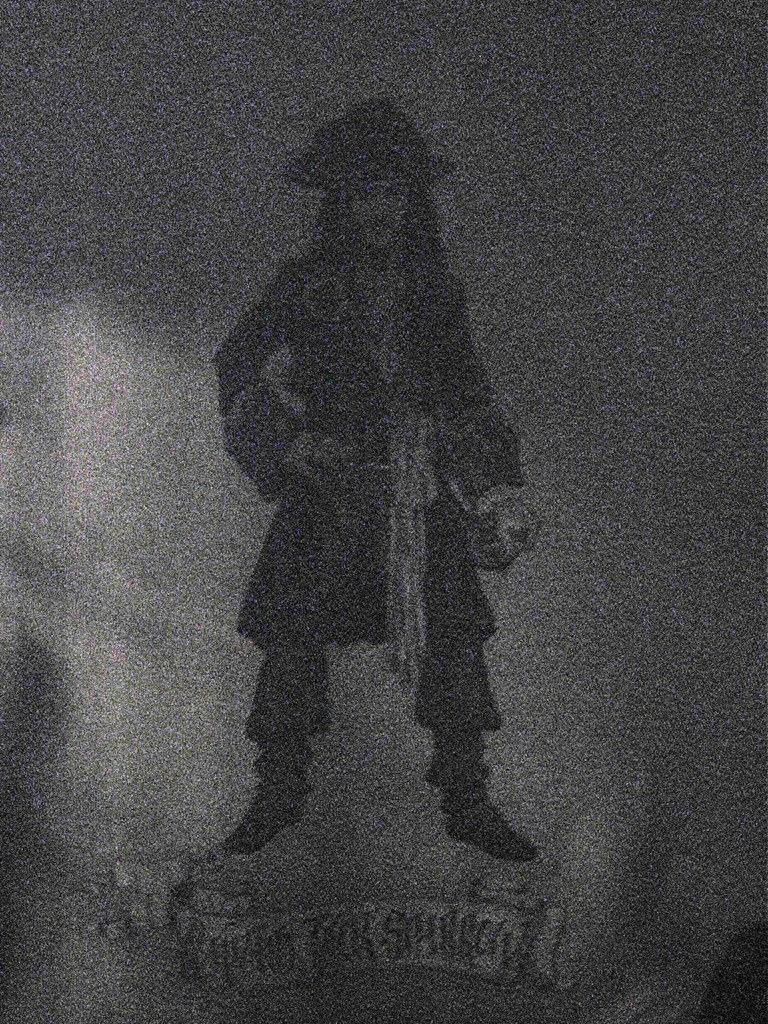The image appears to be an enigmatic and deliberately obscured portrayal of a pirate, potentially resembling either Johnny Depp's Jack Sparrow from "Pirates of the Caribbean" or the iconic figure of Captain Morgan from the rum bottle. Rendered in what looks like charcoal or possibly an intentionally blurred medium, the artwork is enveloped in darkness and ambiguity, reminiscent of an old, fuzzy TV channel.

At the bottom, there's a scroll that seems to bear Latin text, but the words are indiscernible due to the image's heavy obscuration. The pirate at the center features faint, moderate facial details and can be seen wearing a traditional pirate's outfit, complete with a distinctive hat and a buckle on his right shoulder. His left hand clutches an indistinguishable object, while his right hand appears to rest on his belt line or waist.

The background is shrouded in blackness, with a dim light emanating from the left side, offering little illumination or detail. The overall impression is one of vintage mystery, as if viewing an undecipherable scene through the static of a bygone television channel.